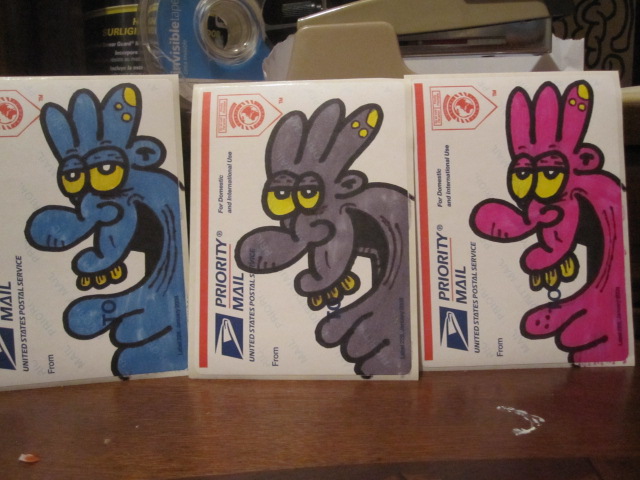The image depicts three USPS Priority Mail envelopes arranged side by side on a brown wooden surface, facing the viewer. Each white envelope features a prominently decorated cartoonish drawing in a vibrant street art style. The characters on the envelopes have a goofy appearance with three buck teeth, yellow eyes, and three tentacle-like prongs on their heads, topped with yellow circles. Their facial features include an open mouth, a long nose, and triple chins, contributing to their quirky demeanor. The characters are the same, but each is colored differently: the leftmost one is blue, the middle one is gray, and the right one is magenta.

The envelopes are adorned with the standard USPS priority mail design, including a yellow border across the top, a blue eagle within a blue square, and "Priority Mail" text accompanied by the United States Postal Service logo. Above the envelopes, one can glimpse the side of a tan stapler and a roll of blue and clear scotch tape. The overall scene captures a playful and creative alteration of everyday postal items.